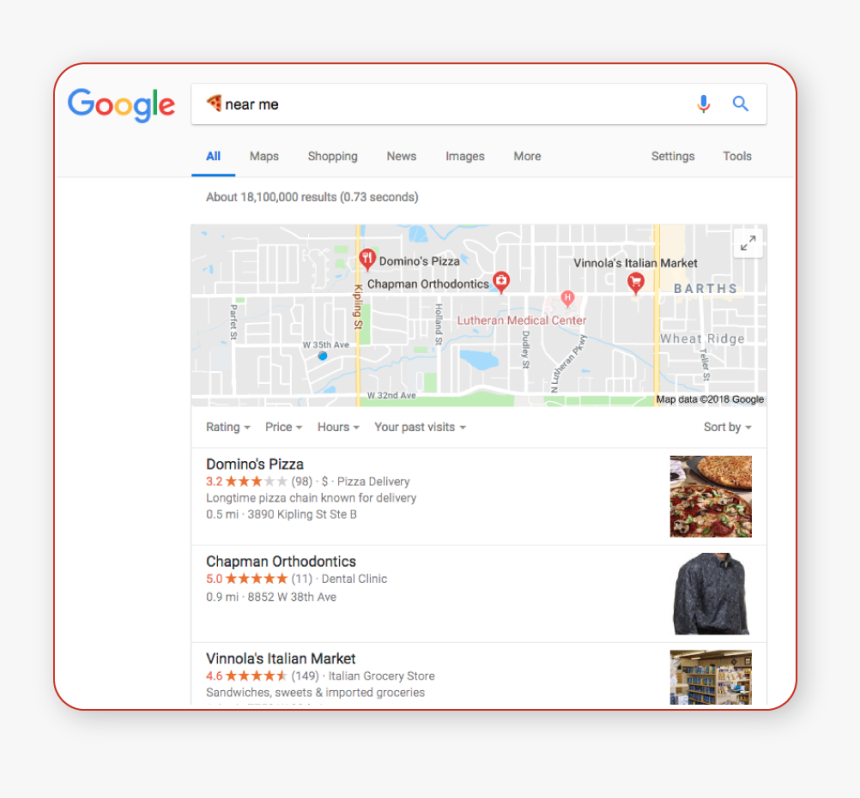The image depicts a Google search results page. At the top, there is a light gray square in the background with a red outlined square featuring rounded corners and a white interior. In the upper left-hand corner of this white space, the word "Google" appears in various colors. Below, a white rectangle with a gray outline contains a picture of a slice of pizza on the left, accompanied by the text "near me." On the right side of this rectangle, there are icons of a microphone and a magnifying glass.

Below the search bar are blue and gray text links, with "All" highlighted and underlined in blue. The other options include "Maps," "Shopping," "News," "Images," "More," "Settings," and "Tools." Directly beneath these links, it states "About 18,100,000 results (0.73 seconds)."

Following this, there is an image of a map with red highlights, followed by filter options including "Ratings," "Price," "Hours," "Your past visits," and a "Sort by" dropdown menu. 

The first search result is for "Domino's Pizza," showing a 3.2 rating with three orange stars and two gray stars. It notes that it is a pizza delivery service, a long-standing pizza chain known for delivery, located 0.5 miles away, followed by an address and a picture of a pizza.

The second result is for "Chapman Orthodontics," rated at 5.0 with all stars filled in orange and the number 11 in parentheses. It is identified as a dental clinic situated 0.9 miles away with an address, and a picture of a man in a black shirt appears on the right.

The final listed result is "Vinola's Italian Market," rated at 4.6 with mostly filled orange stars and the last star partially filled, with the number 149 in parentheses. It is described as an Italian Grocery Store that offers sandwiches, sweets, and imported groceries. A picture of grocery shelves is displayed on the right.